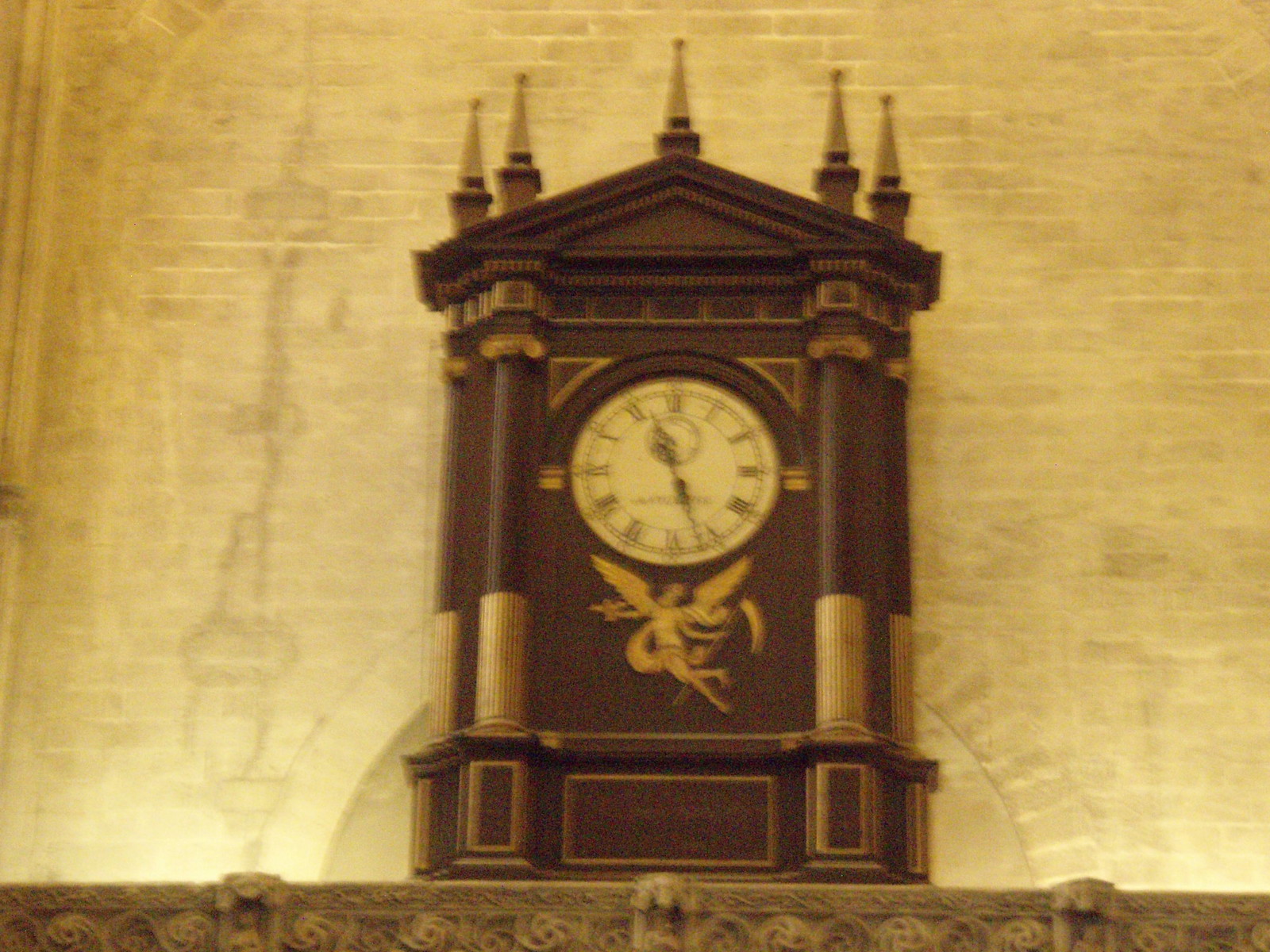A detailed antique clock is prominently placed on a wooden mantle. The background is a yellowish patterned wallpaper that adds a vintage touch to the scene. The clock, which stands approximately a foot and a half tall, features intricate craftsmanship. The front of the clock is adorned with two symmetrical columns flanking the clock face. The clock face itself is cream-colored, with elegant Roman numerals in black, providing a stark and classic contrast. Above the face, a delicate golden figure, resembling a fairy or angel, appears to be in flight. The lower section of the clock is decorated with gold-trimmed paneling, adding an extra layer of ornate detailing. Crowning the clock is a pointed, roof-like structure, embellished with five small steeples, completing its majestic appearance.